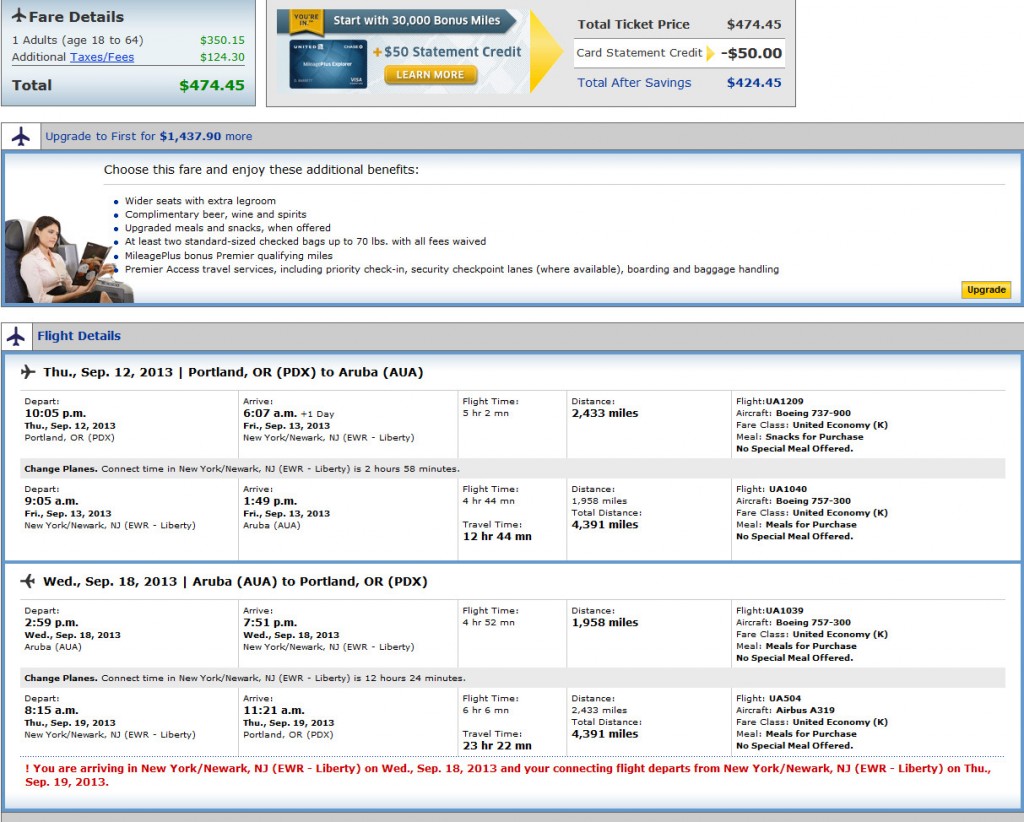A detailed page of flight details and fares.

At the top, the page highlights an offer of 30,000 bonus miles and a $50 statement credit. The standard ticket price is listed as $474.45, but with the $50 credit applied, the total comes to $424.45. There's an option to upgrade to first class for an additional $1,437.90.

Choosing the first-class upgrade provides several additional benefits: 
- Wider seats and extra legroom 
- Complimentary beer, wines, and spirits 
- Upgraded meals and snacks when available 
- At least two standard-sized checked bags up to 70 pounds, with all fees waived 
- MileagePlus bonus premier qualifying miles 
- Premier Access travel services, which include priority check-in, security checkpoint lanes (where available), boarding, and baggage handling

A prominent yellow button allows users to upgrade if they opt to spend the extra amount. Below this section, the page lists various flight options for selection.